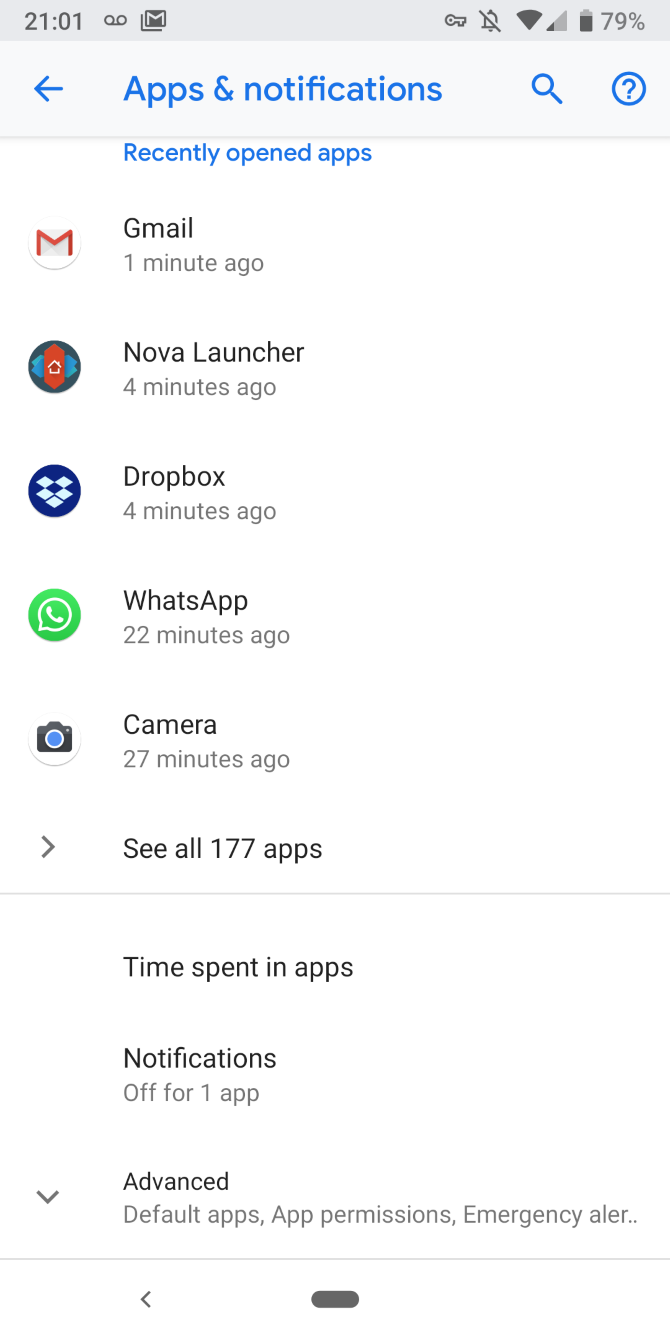A detailed screen capture from a smartphone shows the device set to military time at 21:01, which converts to 9:01 PM in standard time. The battery level is at 79%, and the device has a few bars for internet connectivity. The screen displays a gray banner with blue text titled "Apps and notifications." Users can ask questions or perform searches within this menu. Below the banner, a log of recently opened applications is visible, showcasing the user's activity. 

- **Gmail:** Opened one minute ago with its recognizable logo.
- **Nova Launcher:** Accessed four minutes ago, although its identity is less familiar.
- **Dropbox:** Also opened four minutes ago, hinting at potential back-and-forth usage with Nova Launcher.
- **WhatsApp:** Accessed 22 minutes ago.
- **Camera:** Used 27 minutes ago.

A button is available to view all 177 installed apps, highlighting the extensive number of applications on the device. Additionally, options to see the time spent on each app, view notifications, and access advanced settings are present.